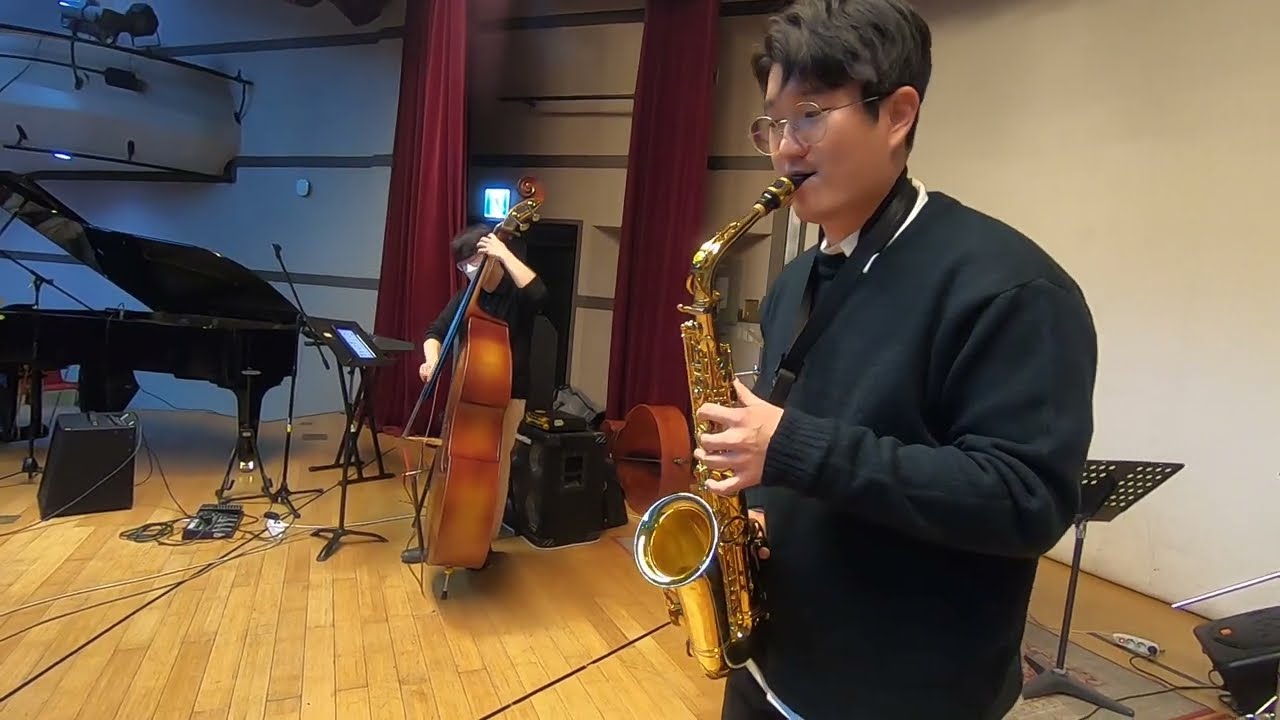In this detailed color photograph, two young Asian males, both around 16 years old, are intensely practicing their musical instruments on a small stage in a modest auditorium. The stage features a brightly yellowish wooden floor and beige-to-white walls. The young man on the left is seated, deeply focused on playing a large cello. He is dressed in a black outfit and is positioned near a grand piano at the left background, which has a stereo in front of it and various wires plugged in around it. On the right side of the image stands another young man, also dressed in a dark jacket over a dress shirt. He has short black hair and wears wire glasses, which accentuate his concentration as he plays a shiny yellow metal saxophone, held by a strap over his shoulder. The saxophonist is facing towards the bottom left corner of the image. Behind him, one can also spot a bass on a stand and a couple of black music stands. This photograph, characterized by its realistic and representational style, suggests a quiet moment of dedicated practice, with no other people in sight, emphasizing the duo’s earnest effort and commitment to their musical craft.